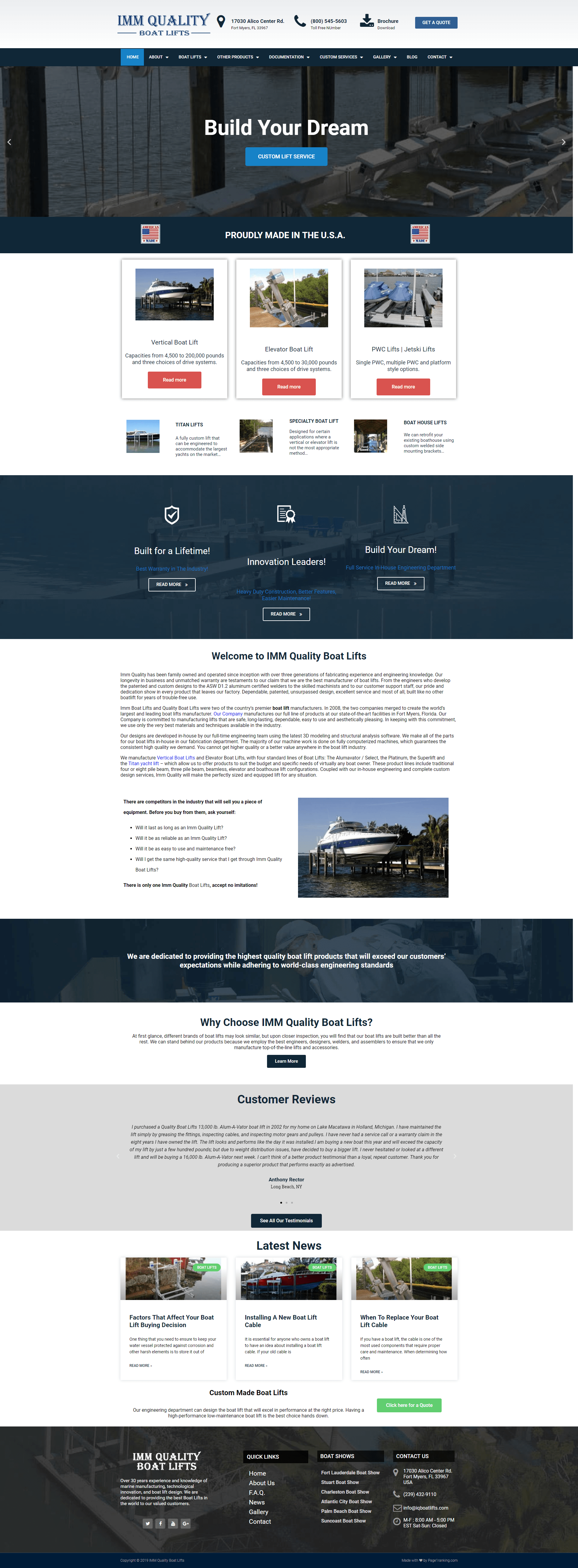IMM Quality Boat Lifts, located at 17030 Alico Center Road, offers a comprehensive product overview and services on their website. Here, visitors can download a detailed brochure or request a quote using a prominent blue button. The site features a striking photo with the tagline "Build Your Dream," highlighting their "Custom Lift Service" which is proudly made in the USA. 

Above this main section, the navigation menu is organized into several categories including: Home, About, Boat Lifts, Other Products, Documentation, Custom Services, Gallery, Blog, and Contact, each with a drop-down menu for more options. 

Directly below the main photo, three boxed images showcase different types of lifts: vertical boat lifts, elevator boat lifts, and PWC (Jet Ski) lifts, each with a “Read More” link for additional information. Further down, additional categories such as Titan Lifts, Specialty Boat Lifts, and Boat House Lifts are listed, emphasizing their durability and innovative design under slogans like "Built for Life" and "Innovative Leaders."